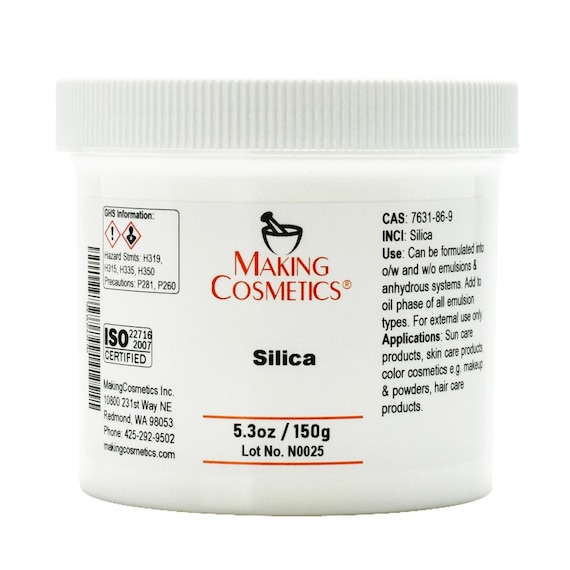The image features a white jar set against a plain white background. The jar has a lid with numerous vertical indentions and a prominent red band around its center. In the middle of the lid, "Making Cosmetics" is boldly printed in red capital letters, accompanied by a simple line art illustration of a bowl with a utensil inside. Directly beneath this, the word "Silica" is displayed in black lettering. A thin horizontal red line both above and below frames the text, with the statement "5.3 oz / 150 g" located between these lines. Below this, the lot number "N0025" is inscribed in black letters. Additional details extend to the sides of the jar, including a column of text on the left side with use instructions, applications, and the CAS number "7631-86-9" and INCI name "silica." This side text specifies that the silica can be formulated in O/W emulsions and anhydrous systems, and should be added to the oil phase of all emulsions. The product is also noted to be ISO certified, with warning labels and a UPC barcode included in the design.